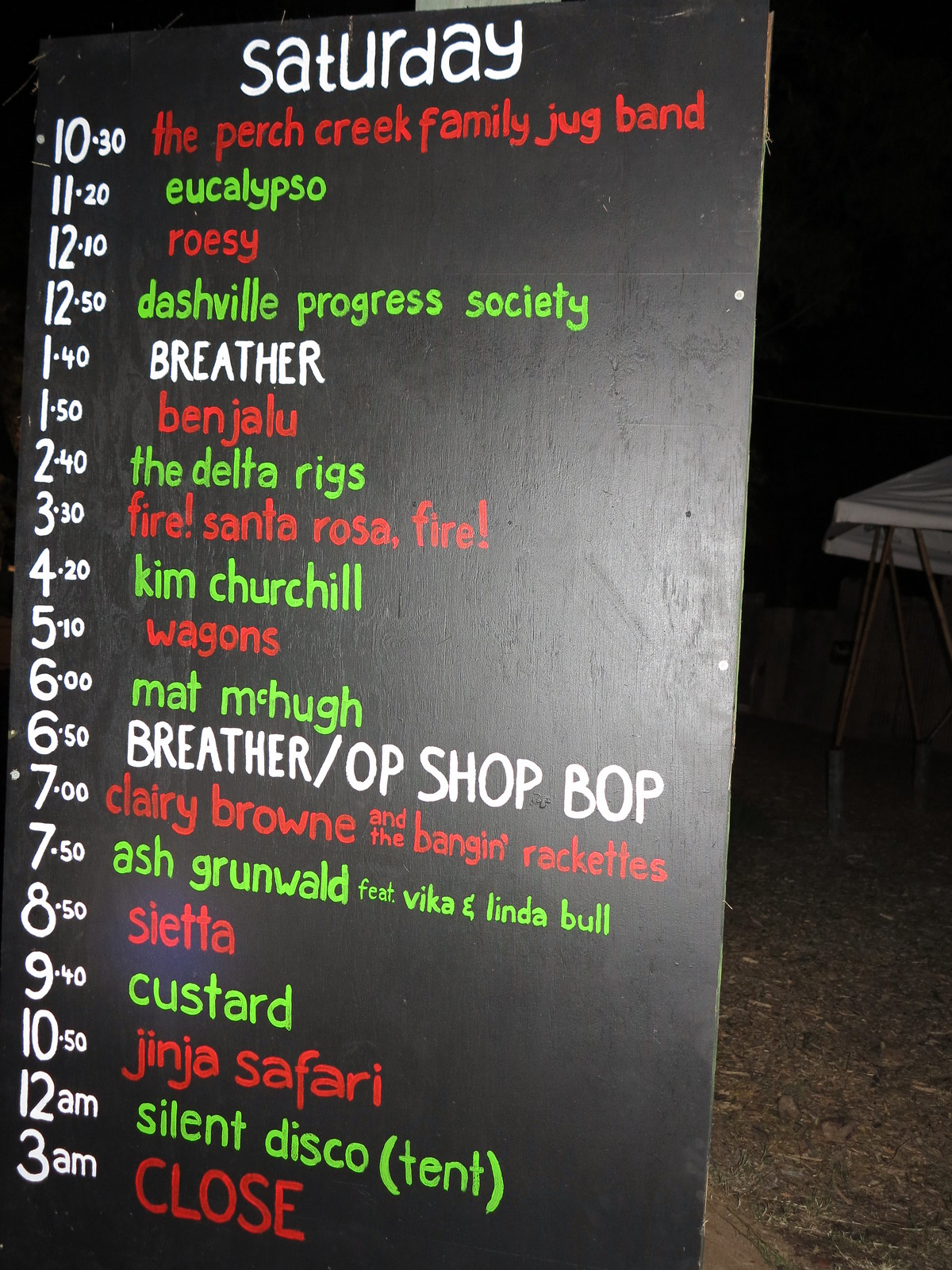This image is a color photograph in portrait orientation, featuring a detailed schedule of musical acts written on a blackboard with red, green, and white lettering. At the top, "Saturday" is written in white. The schedule begins at 10:30 AM with "The Perch Creek Family Jug Band" in red. Following this at 11:20 AM is "Eucalyptso" in green, and at 12:40 PM, "Rosie" in red. The "Dashville Progress Society" appears at 12:50 PM in green, followed by "Breather" at 1:40 PM in white. "Benjalou" is listed at 1:50 PM in red, and "The Delta Rigs" at 2:40 PM in green. At 3:30 PM, "Fire! Santa Rosa, Fire!" is highlighted in red. "Kim Churchill" is scheduled for 4:20 PM in green. "Wagons" perform at 5:10 PM in red, followed by "Matt McHugh" at 6:00 PM in green. At 6:50 PM, "Breather / O.P. Shop Bop" are mentioned in white. "Clary Brown and the Bangin' Rackettes" are listed at 7:00 PM in red. "Ash Grunwald featuring Vika and Linda Bull" appear at 7:50 PM in green, with "Custer" at 8:50 PM also in green. "Jinja Safari" is scheduled for 10:50 PM in red. The evening concludes with a "Silent Disco Tent" at 12:00 AM in green, and the event closes at 3:00 AM in red. The placement of times on the left side and the colorful writing suggests a vibrant and organized event.